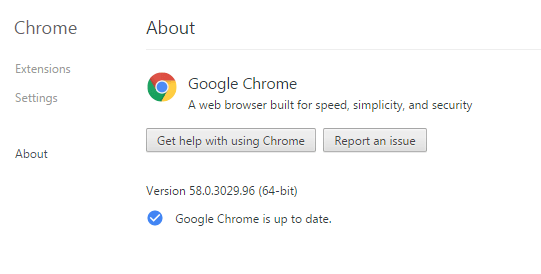The screenshot captures a Google Chrome settings page displayed on a computer desktop with a predominantly white background. At the top of the image, "Chrome" is faintly written in black text. Beneath this title, there are menu options: "Extensions" and "Settings" in grey ink, and "About" in faint black ink, indicating that the "About" section is currently selected.

On the right side of the screen, the Google Chrome logo is prominently displayed, followed by the description: "Google Chrome: a web browser built for speed, simplicity, and security," written in black text. Below this description, there are two clickable options: "Get help with using Chrome" and "Report an issue," both in black text on grey background tabs.

The screenshot also shows the current version of Google Chrome along with a message stating "Google Chrome is up to date," accompanied by a white tick inside a blue circular background.